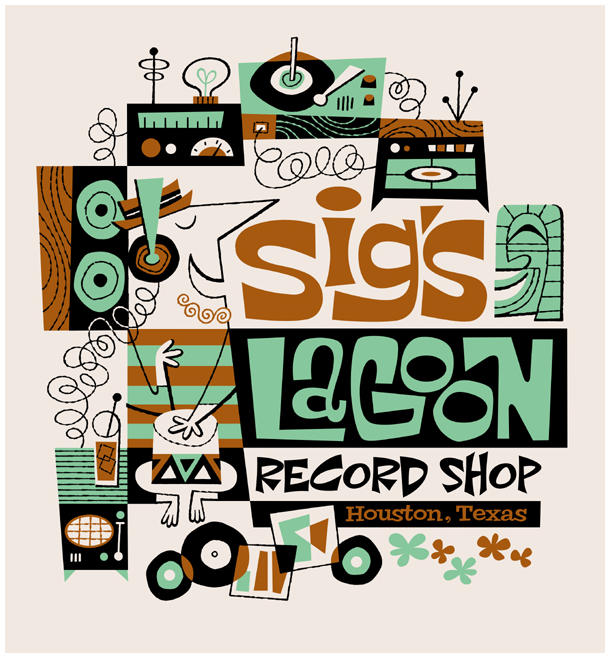The advertisement displays a retro-themed poster for Sig's Lagoon Record Shop located in Houston, Texas. The poster embodies a distinct mid-century aesthetic, reminiscent of the late 50s and early 60s, featuring a soothing palette of pale greens, browns, and light tan backgrounds. Dominated by geometric shapes evocative of the era, the design includes circles and rectangles that create imagery suggestive of turntables, records, and speakers. 

Centrally placed yet slightly off to the right, the text commands attention with "SIG'S" in prominent brown text, followed by "Lagoon" in green lettering within a black rectangle, and "Record Shop" beneath it in black ink. "Houston, Texas" is inscribed below in brown. A beatnik-styled illustration of a man playing bongos with a squiggly beard adds character, harking back to the tiki culture. Other visual elements include a record player, a radio, speakers, records on the floor, and a record table with a hi-fi system, accentuated with flower petal designs and black curly cables, further enhancing the nostalgic vibe.